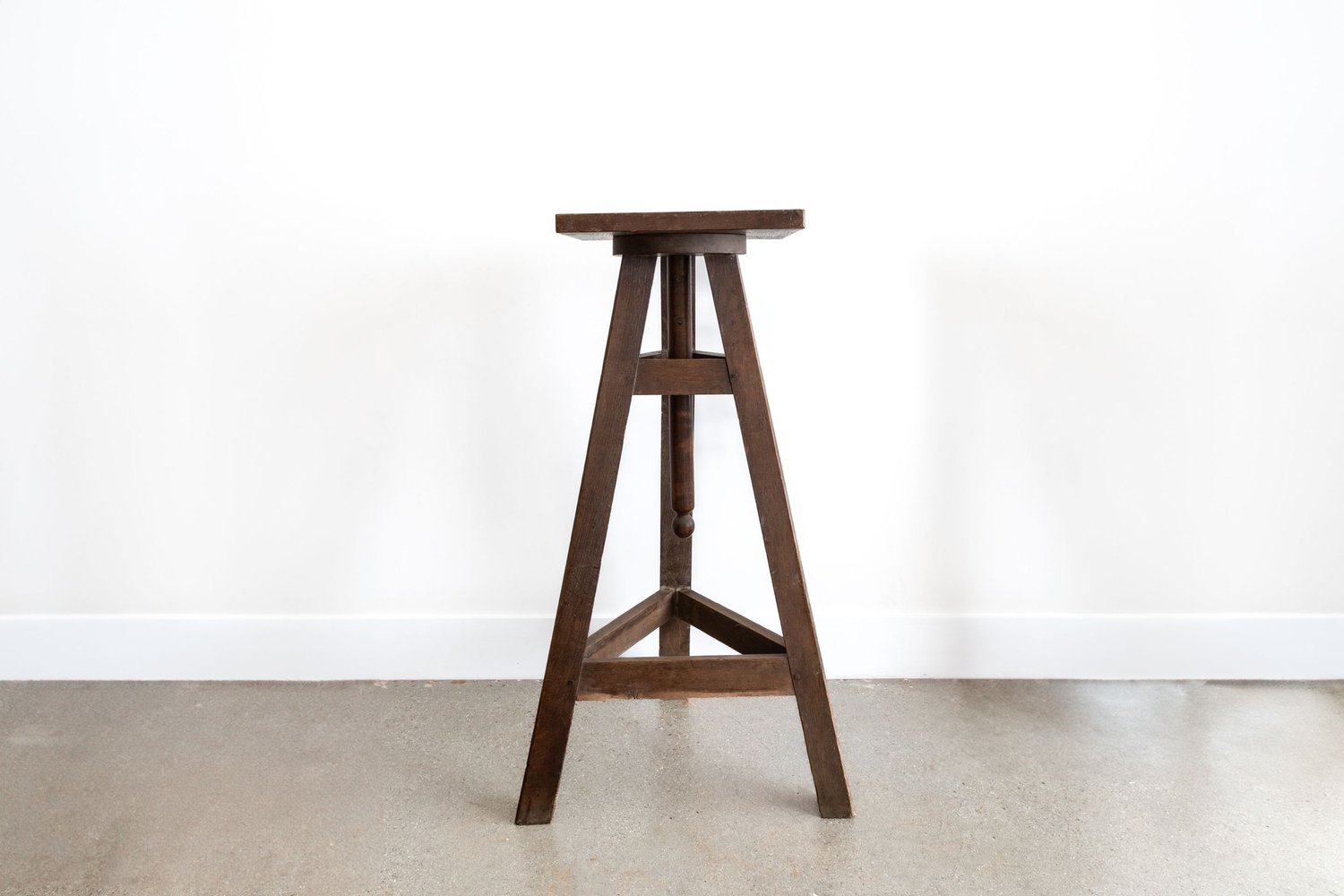The photograph captures a dark wood barstool with a square top, positioned against a solid white wall in a room with a light gray and beige floor, potentially made of stone or wood. The barstool’s distinctive design features three legs, resembling a tripod, with triangular supports both a quarter of the way down from the top and a quarter of the way up from the bottom. Notably, there is a central wooden beam extending downwards from the seat, contributing to its structural integrity. The clean, minimalist setup accentuates the stool's dark brown, possibly oak finish against the neutral-toned backdrop.